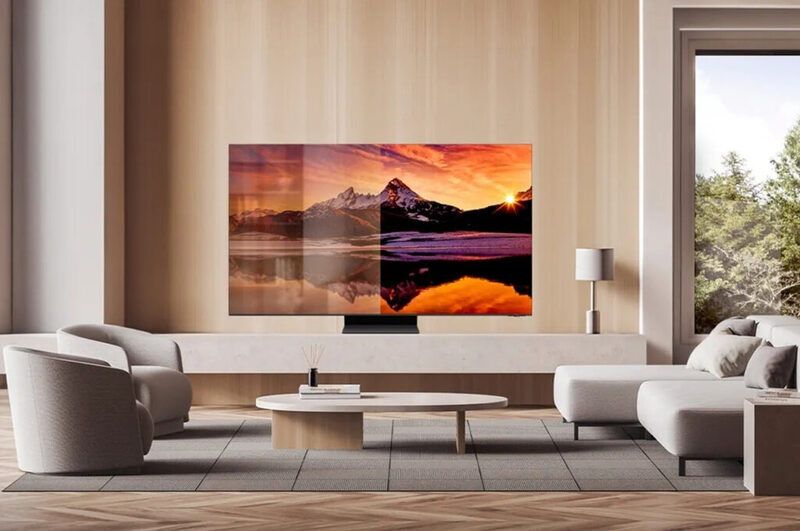This indoor color photograph captures a spacious, modern living area with a minimalistic design. The room features neutral tones, with light tan walls and cream-colored furniture, including two small round chairs, a chaise lounge, and a wide chair, some of which may be connected. A minimalistic round coffee table with a unique design, displaying a book and a diffuser, is situated in the midst of the seating arrangement.

The focal point of the image is a very large flat-screen TV centrally located, vividly displaying a sunlit mountain range at sunset, with the mountains beautifully reflected in a lake in the foreground. To the right of the TV is a cream-colored lamp, and further right, a window offers a view of greenery and a blue sky, ensuring the minimalist decor remains visually calm and serene. The striking contrast of vibrant colors on the TV screen against the subdued tones of the room highlights the television as the central element of this tranquil and elegantly designed living space. Notably, there are no people in the image, emphasizing the serene, unoccupied ambiance.